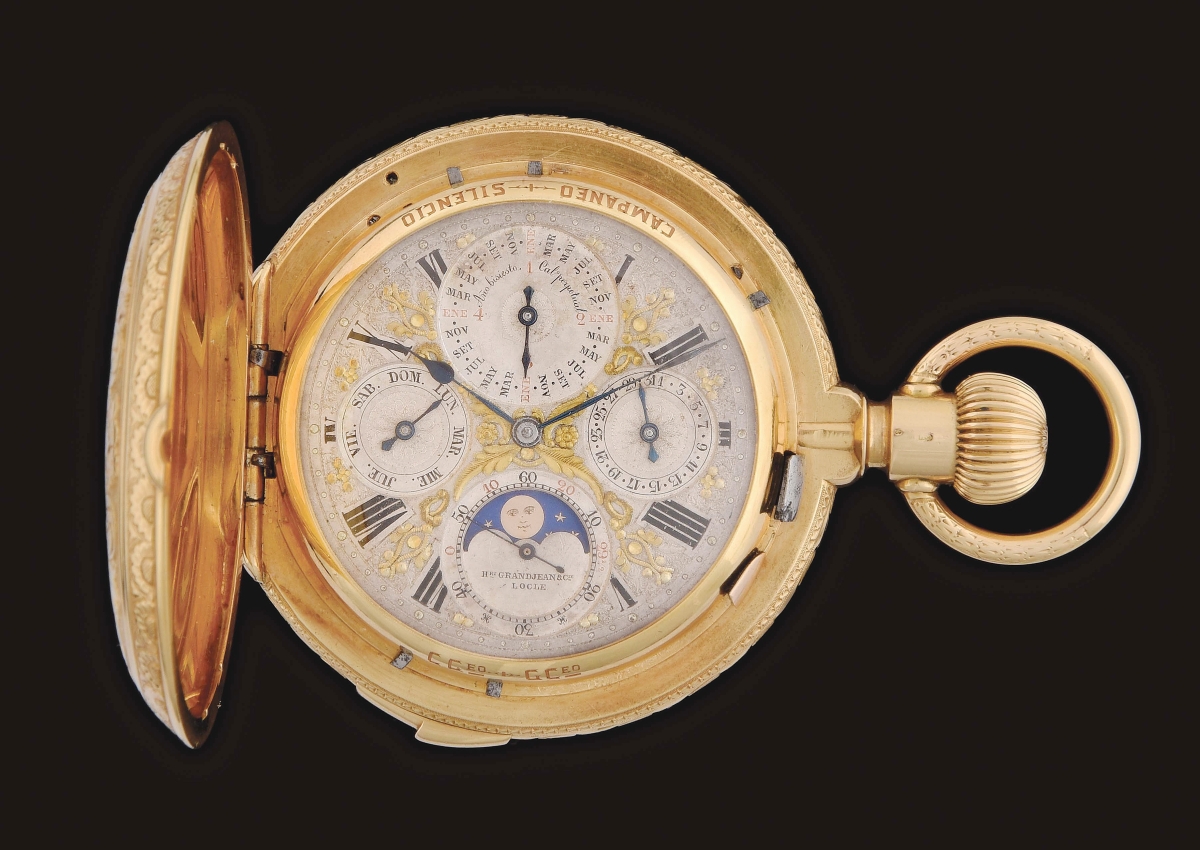The professionally staged, full-color photograph features a golden antique pocket watch suspended against a stark black background. The square image showcases the watch with its ornate lid open, revealing intricate etching on both the exterior and interior. The cover's hinge is positioned to the left side of the watch, highlighting a ring and a winding crown on its right. 

Inside, the watch face is a contrasting white, adorned with four distinct dials. The main face, marked by Roman numerals, features two central gray hands indicating the hours and minutes. The uppermost dial is a calendar displaying the months of the year. The bottom dial portrays a moon and stars, likely indicating lunar phases. The other two dials are positioned on the left and right sides of the watch face. The left dial measures the date, while the right dial's specifics are unclear but might include degrees and possibly the year. Above these dials, at the top of the watch face, is the text "Impaigned Silence," rendered upside down.